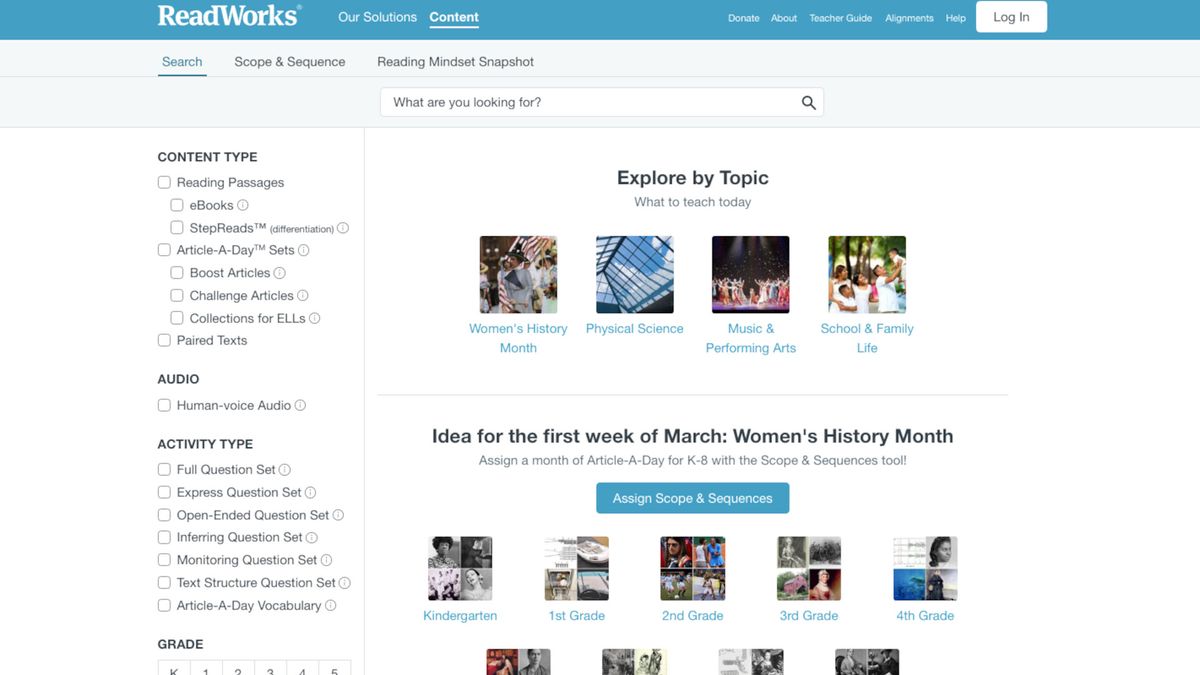In this screenshot, we see the homepage of Readworks, marked by a blue banner running horizontally across the top as the header. The company's name, "Readworks," is prominently displayed in bold white block text on this banner. To the right, a navigation menu lists the options: Our Solutions, Content, Donate, About, Teacher Guide, Alignments, and Help, followed by a white login button.

Beneath the header, a secondary navigation bar includes options for Search, Scope and Sequence, and Reading Mindset Snapshot. A white search bar sits just below this, containing placeholder text reading "What are you looking for?" beside a gray magnifying glass icon.

The middle section of the screenshot features a bolded title, "Explore by Topic," followed by a segment labeled "What to Teach Today." This area showcases four square color images, each representing a different topic. The first image highlights "Women's History Month," the second focuses on "Physical Science," the third depicts "Music and Performing Arts" with several performers on a stage under spotlights, and the fourth image, titled "School and Family Life," portrays a family of five standing outdoors, composed of three children and their parents.